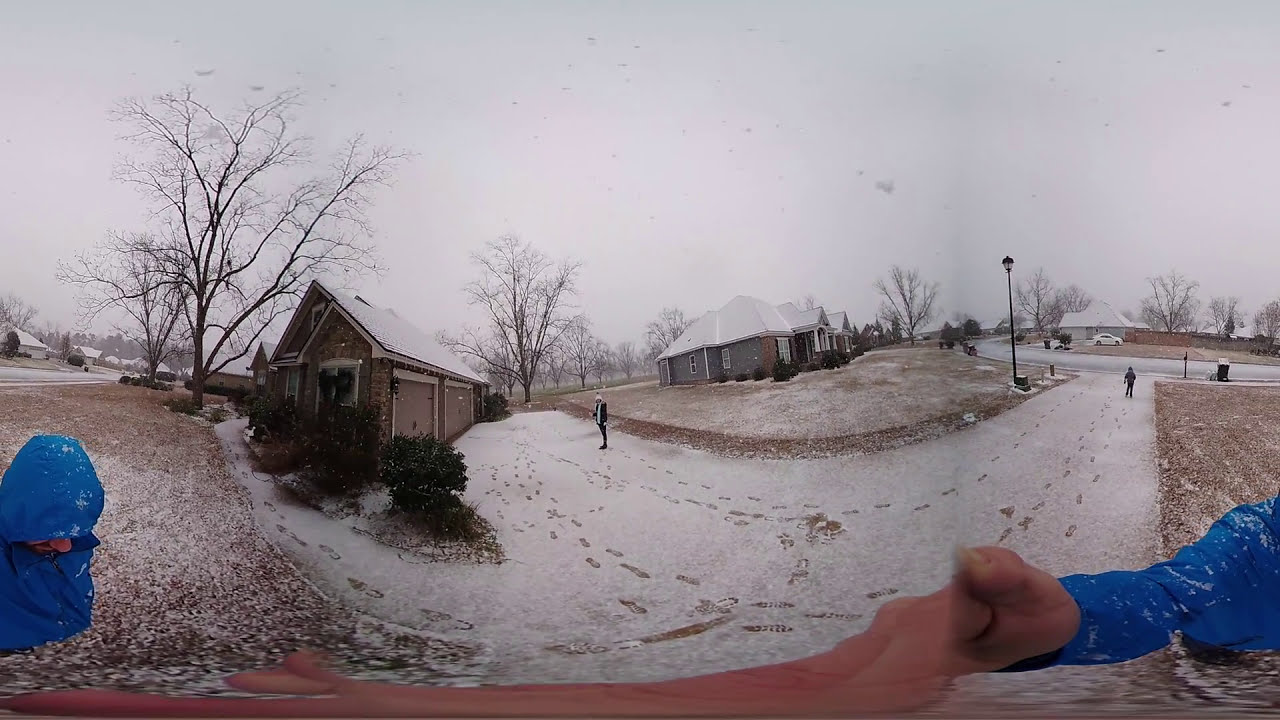A panoramic first-person perspective captures a snowy outdoor scene with a driveway leading to a light brown brick house on the left, featuring two garages and two snow-covered triangular roofs. The thin layer of snow on the ground reveals multiple footsteps forming a U-shaped track. To the left of the U's end, evergreen shrubs line the front of the house. The road extends from the center left to the right, bordered by additional snow-dusted houses and leafless trees. The overcast sky appears grey-white. The photographer, wearing a blue coat with a hood, is visible in the bottom left, their elongated arm stretches across the bottom of the image due to the panorama stitching. Two other people, dressed in black, are seen standing on the driveway, one straight ahead and another to the far right. Snow is also visible on the photographer’s hood and sleeve.